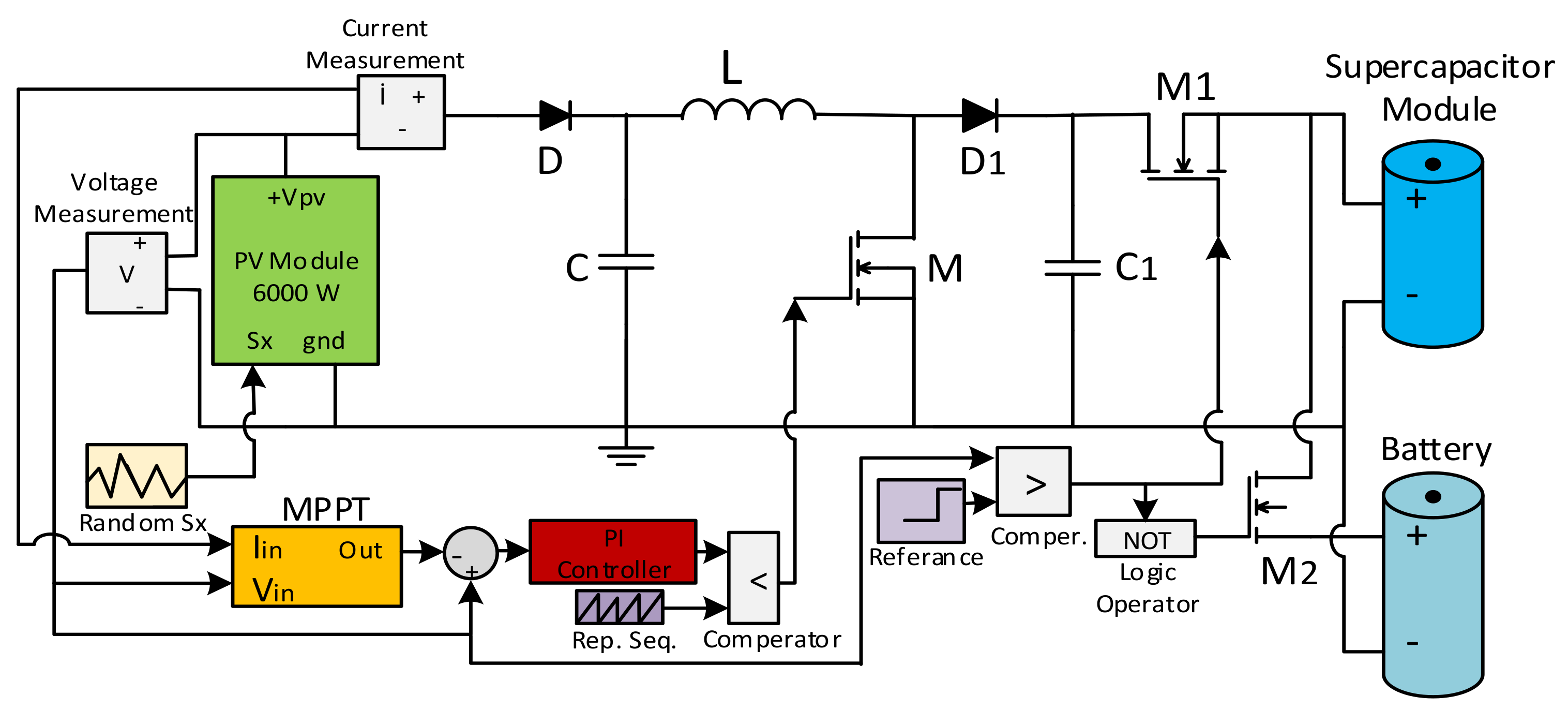This intricate diagram is an electrical circuit schematic presented on a white background, showcasing various interconnected components and measurements. Predominantly rendered in black text and lines, the image employs different colors to highlight larger boxes and specific elements. Central to the diagram are the symbols and arrows indicating the flow of current and voltage. 

At the heart of the schematic, a green rectangular box denotes a 6000-watt PV module, with associated inputs and outputs clearly marked. Nearby, gray squares labeled "current measurement" and "voltage measurement" highlight crucial monitoring points within the circuit. Further along, the diagram features a sequence of colored rectangles, including an orange one marked "in, out, in," leading through various elements to a red rectangle labeled "PI controller."

On the right side of the schematic, two cylinders represent energy storage units: a dark blue supercapacitor module positioned above a lighter blue battery. Additional components such as logic gates, comparators, and various ground connections (noted as "5x GND plus VPV") are intricately detailed, collectively forming a comprehensive and complex electrical plan.